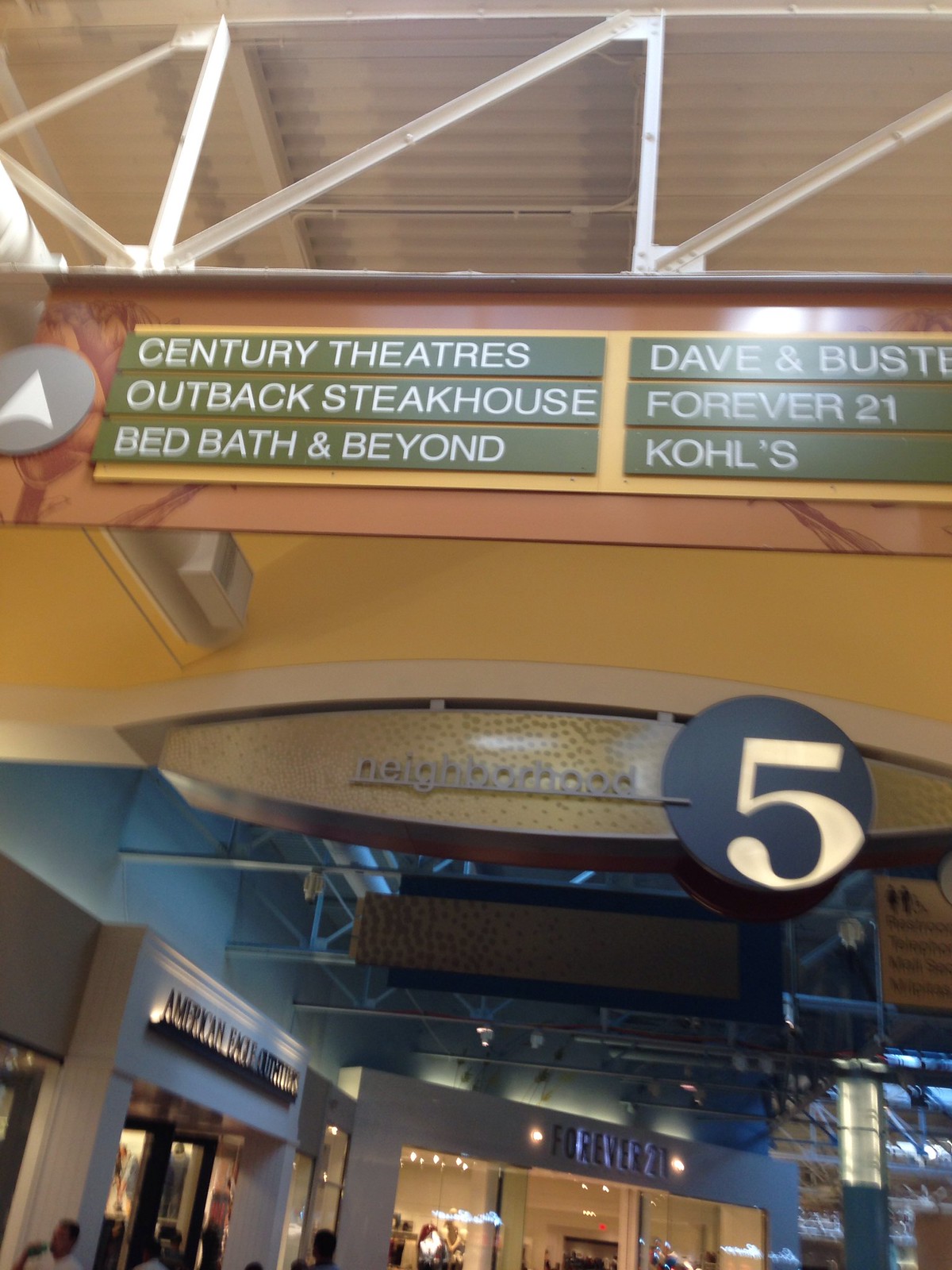This photo, taken inside a bustling mall, captures the industrial-style ceiling adorned with metal bars extending down towards a prominent directional sign. The sign is divided into several green rectangles with white lettering, guiding visitors to various stores: Century Theatres (accompanied by a white arrow and grey circle), Bed Bath & Beyond, Dave & Buster's, Forever 21, and Kohl's. Beneath this sign, attached to the wall, is another sign with grey lettering that reads "Neighbourhood 5" – the number 5 is inside a navy circle with white digits. In the background, framed by the structural elements of the mall, are recognizable storefronts for American Eagle Outfitters and Forever 21, hinting at the vibrant retail environment of the location.